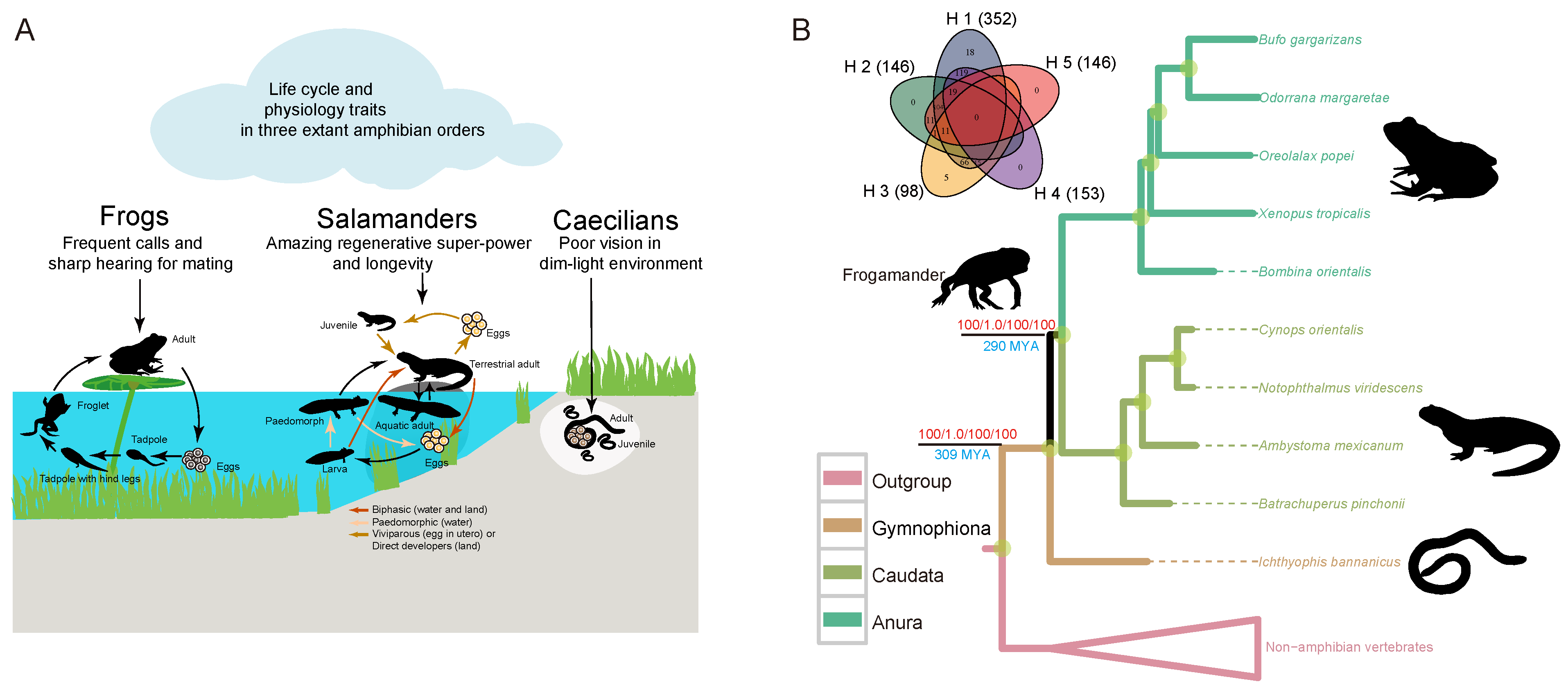The image consists of two distinct diagrams, labeled A (left) and B (right), both illustrating various aspects of amphibian life cycles and related traits. Diagram A is set against a white background with a light blue cloud at the top, containing the title "Life Cycles and Physiology Traits in Three Extant Amphibian Orders" in black text. The diagram displays life stages and physiological details of frogs, salamanders, and caecilians. On the left side, there is a series of black silhouettes showing the frog's life stages, starting with eggs in blue water, transitioning through a tadpole, tadpole with hind legs, immature frog, and finally, an adult frog sitting on a lily pad surrounded by green grass. It highlights features such as "frequent calls" and "sharp hearing for mating."

Adjacent to this, the salamander's life cycle is depicted, starting with eggs, progressing through various stages including larvae, juvenile, and adult phases. The text emphasizes the salamander's "amazing regenerative superpower and longevity." Finally, the caecilian's life stages are depicted with eggs and juvenile stages shown in a dim, underground environment, emphasizing "poor vision in dim-lit environments."

On the right, Diagram B delves into the taxonomy and evolutionary relationships among these amphibians. It features a complex, color-coded star-shaped diagram with various numbers and letters indicating different classifications and traits. Colors such as red (e.g., H5) and purple (e.g., H4) annotate specific groups and characteristics. A bracketed system shows the evolutionary pathway among frogs, salamanders, and caecilians, summarizing their phylogenetic relationships and their classification into different orders, highlighted in terms of colors representing their grouping (e.g., pink for outgroup, orange for Gymnophiona).

Together, the two diagrams comprehensively describe the life cycles of these amphibians, their physiological traits, and their evolutionary relationships, providing a detailed visual synopsis of amphibian biology and taxonomy.